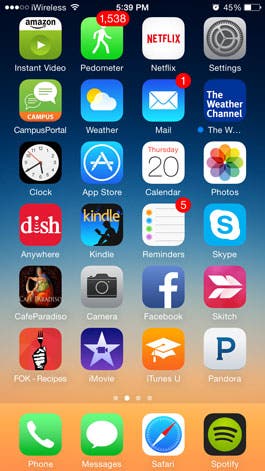This is an image of a cell phone screen displaying a variety of app icons and system information. 

In the top left corner, the screen shows "Wireless" next to a wireless signal icon, with the time displayed as "5:39 PM." In the top right corner, the battery status indicates 45% with an accompanying battery icon.

Beneath this status bar, the home screen features a grid layout with six rows of app icons, each row containing four apps:

1. **Top Row:** Instant Video, Pedometer, Netflix, Settings
2. **Second Row:** Campus Portal, Weather, Mail, The Weather Channel
3. **Third Row:** Clock, App Store, Calendar, Photos
4. **Fourth Row:** Anywhere, Kindle, Reminders, Skype
5. **Fifth Row:** Café Paradiso, Camera, Facebook, Skitch
6. **Bottom Row:** Fox Recipes (assuming "FOK" might be "Fox"), iMovies, iTunes U, Pandora

At the very bottom of the screen, there's a dock with four icons:
- **Phone:** A green box with a phone icon
- **Messages:** A speech bubble icon
- **Safari:** A compass icon
- **Spotify:** The Spotify logo

Overall, the home screen is fully occupied by a diverse selection of applications, neatly organized in a consistent grid pattern.